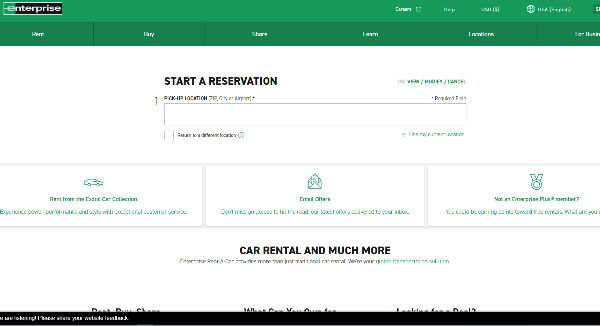This image depicts the home page of the Enterprise Rent-A-Car website. The top section features a green navigation bar with the word "Enterprise" prominently displayed in white font on the left side. On the right side of this bar, there are some partially obscured text elements due to poor resolution.

Below this, another green navigation strip spans across the page. On the left side, it includes menu options beginning with "Home," followed by several indistinct or cut-off items that may include "Store," "Learn," and other options.

The central portion of the page has a white background and focuses on service options. Keytext elements include "Start a Reservation" prominently displayed at the top. Below this, options such as "View," "Modify," and potentially "Cancel" are listed. There's a Pickup Location field with accompanying data input areas that are currently blank. Additionally, a checkbox is present with unclear labeling.

Further down the page, promotional sections are evident: one that mentions obtaining something from the domestic car collection, another possibly referring to a credit offer, and a third area that seems to be associated with Enterprise Plus membership. At the very bottom of the white section, the text reads "Car Rental and much more."